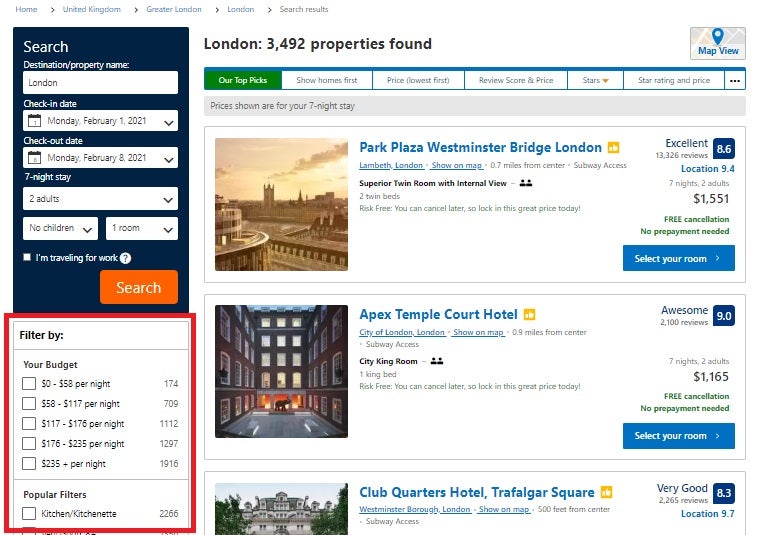The screenshot captures a portion of a travel itinerary website, with the header missing, focusing on the body of the webpage. 

On the left side, there is a search box with a navy blue background and a prominent red "Search" button. This search box allows users to select their destination, choose check-in and check-out dates, specify the number of adults, children, and rooms, and includes an option to indicate if they are traveling for work.

Below the search box, there is a "Filter By" section, encased within a red border. This section features budget filters with five checkboxes for different price ranges per night: 
- $0-$58 
- $58-$117 
- $117-$176 
- $176-$235 
- $235+

Each budget filter shows the number of hotel rooms that fall within the specified price range. Additionally, under "Popular Filters," options such as kitchen and kitchenette are available, along with the number of lodgings that offer these amenities.

The right pane, which is the largest section, displays search results. At the top, it states "London" and indicates that there are 3,492 properties found. The listings for properties appear as separate boxes:

1. **Park Plaza, Westminster and Bridge** 
   - Overall Rating: 8.6
   - Details: Accommodation dates, nights, number of adults, and total amount with a "Select Your Room" blue button.

2. **Apex Temple Court Hotel**
   - Overall Rating: 9

3. **Club Quarters Hotel, Trafalgar Square**
   - Overall Rating: 8.3

Each property listing includes an overall rating, a separate rating for the location, accommodation details including the number of nights and adults, subtotal costs, and a blue "Select Your Room" button.